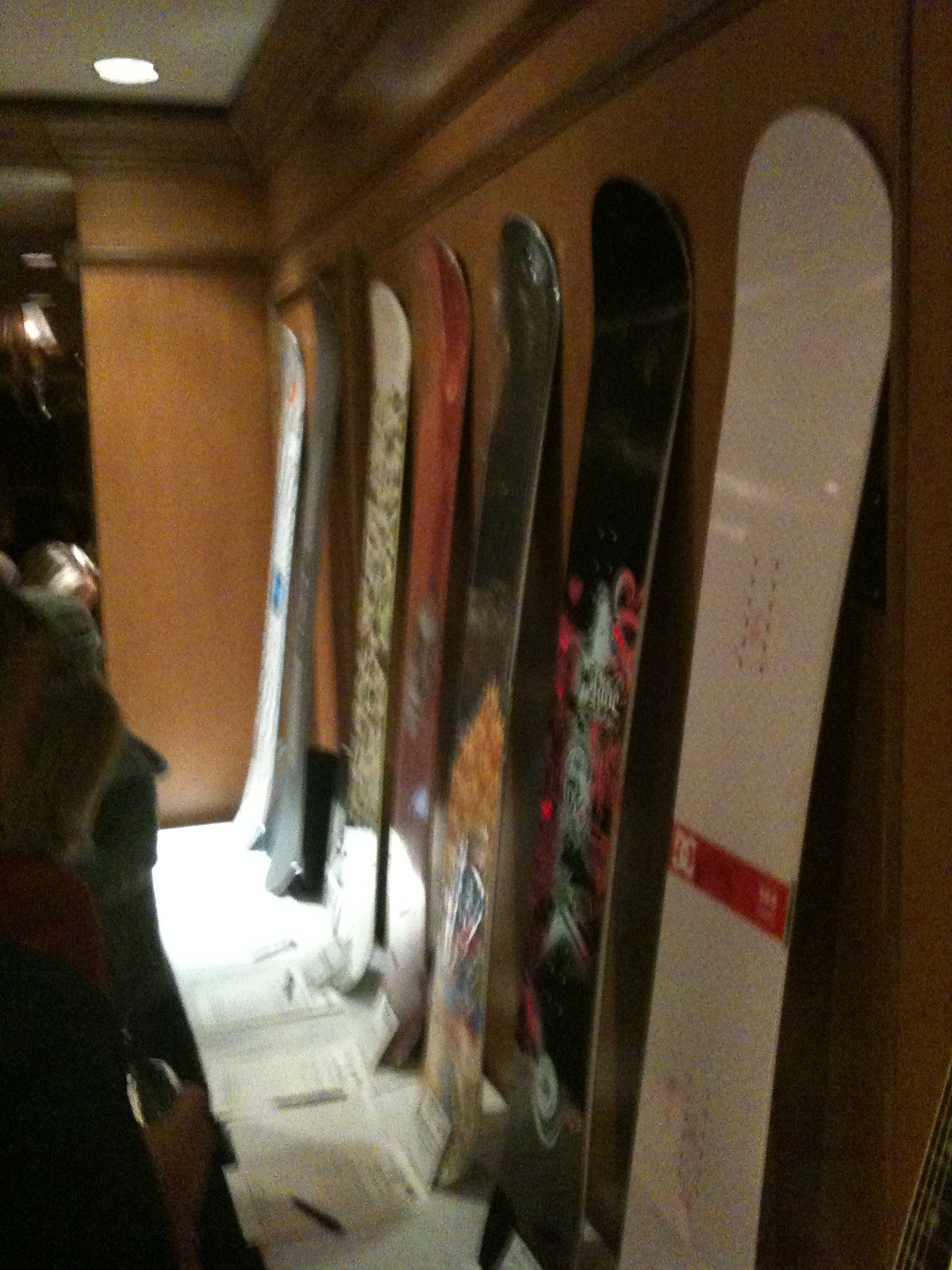The image is a blurry color photograph depicting a dimly lit interior room with rich, dark wood paneling on the walls and a white floor. Overhead, there is a recessed light fixture in the upper left corner of the frame, casting a limited amount of illumination. Additional light spills into the scene from the left side of the frame, brightening the lower portion of the photo. Against the wood-paneled wall, seven snowboards are standing vertically. The snowboards vary in color and design: the one in the foreground is predominantly white with a red band and red lettering across the middle. Two of the snowboards are mainly black, one featuring fiery and skull designs. Another snowboard is glossy black with an orange design. There are also a few white and more colorful, decorated boards further in the background. The floor appears scattered with some kind of paperwork, adding to the room's somewhat cluttered ambiance. Overall, the room gives the impression of being a showroom, a high-end storage area, or an extravagantly outfitted walk-in closet.